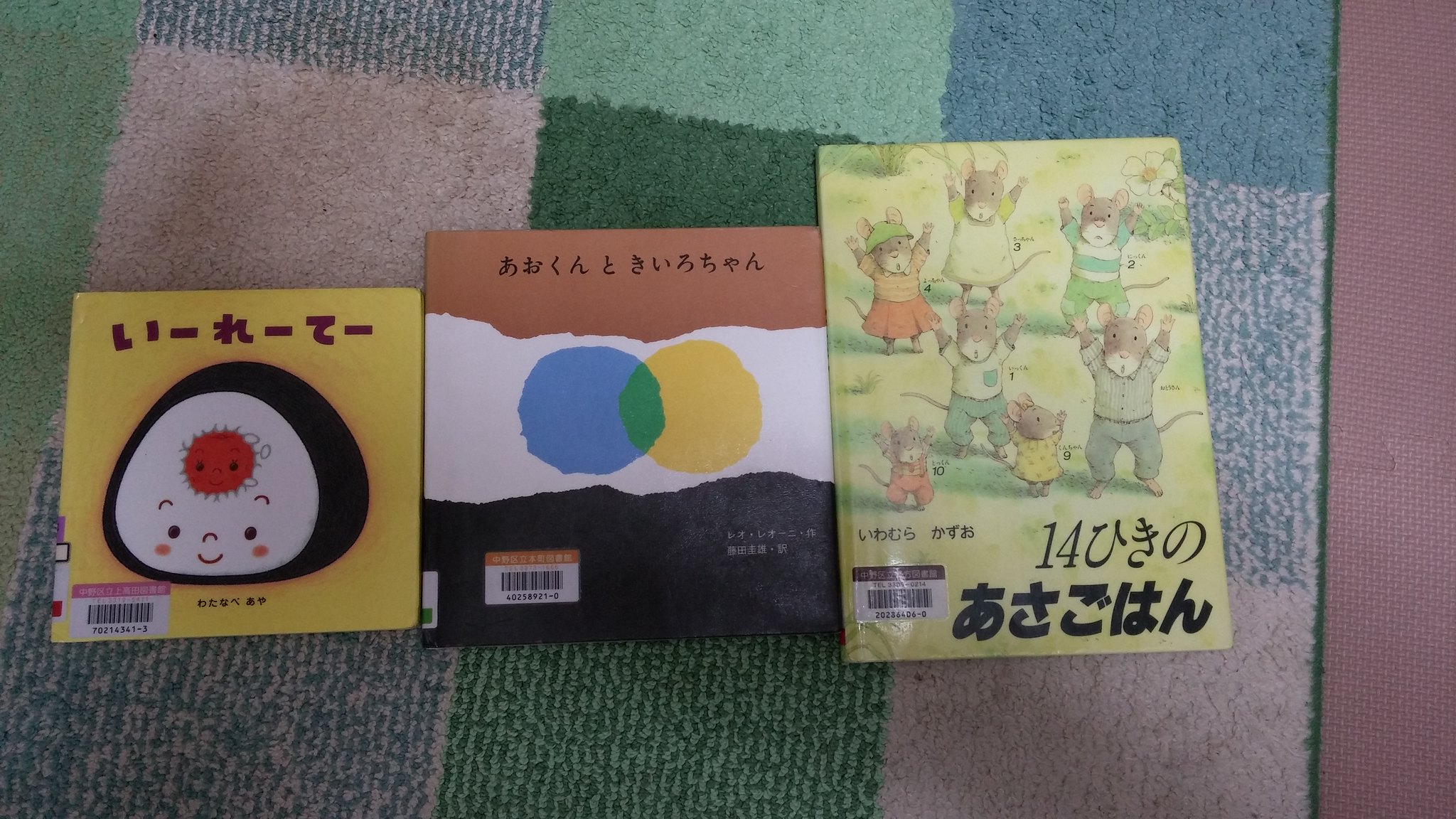The image features three children's books placed on a multicolored, patterned rug, which resembles a patchwork or bath mat. The rug showcases an array of colors, including pink, various shades of green, blue, light lavender, and teal, with tiles that appear striped and dotted. On the far right of the rug, there’s a vertical strip that looks like it has a yoga mat texture in a pink color.

The first book on the left, which is yellow, shows a smiling face of a cartoon character, possibly resembling a baby. This book appears to be written in an Asian language, potentially Mandarin, Japanese, or Korean, and it has a barcode on the front. 

The second book, centrally placed, has a brown border with a white center. It features two interlocking circles, colored blue and yellow, which merge to form green in the middle, and has a black border along the bottom. This book also contains text in a similar Asian script and includes a barcode.

The third book, on the right, depicts a scene with several small animated characters—mice, and possibly bears and bunnies—standing in a green field with their hands raised, expressing surprise or excitement. This book too is in an Asian language and has a barcode on the cover. 

In summary, the image captures a detailed scene of three Asian-language children’s books set against a vividly colored, patchwork rug.